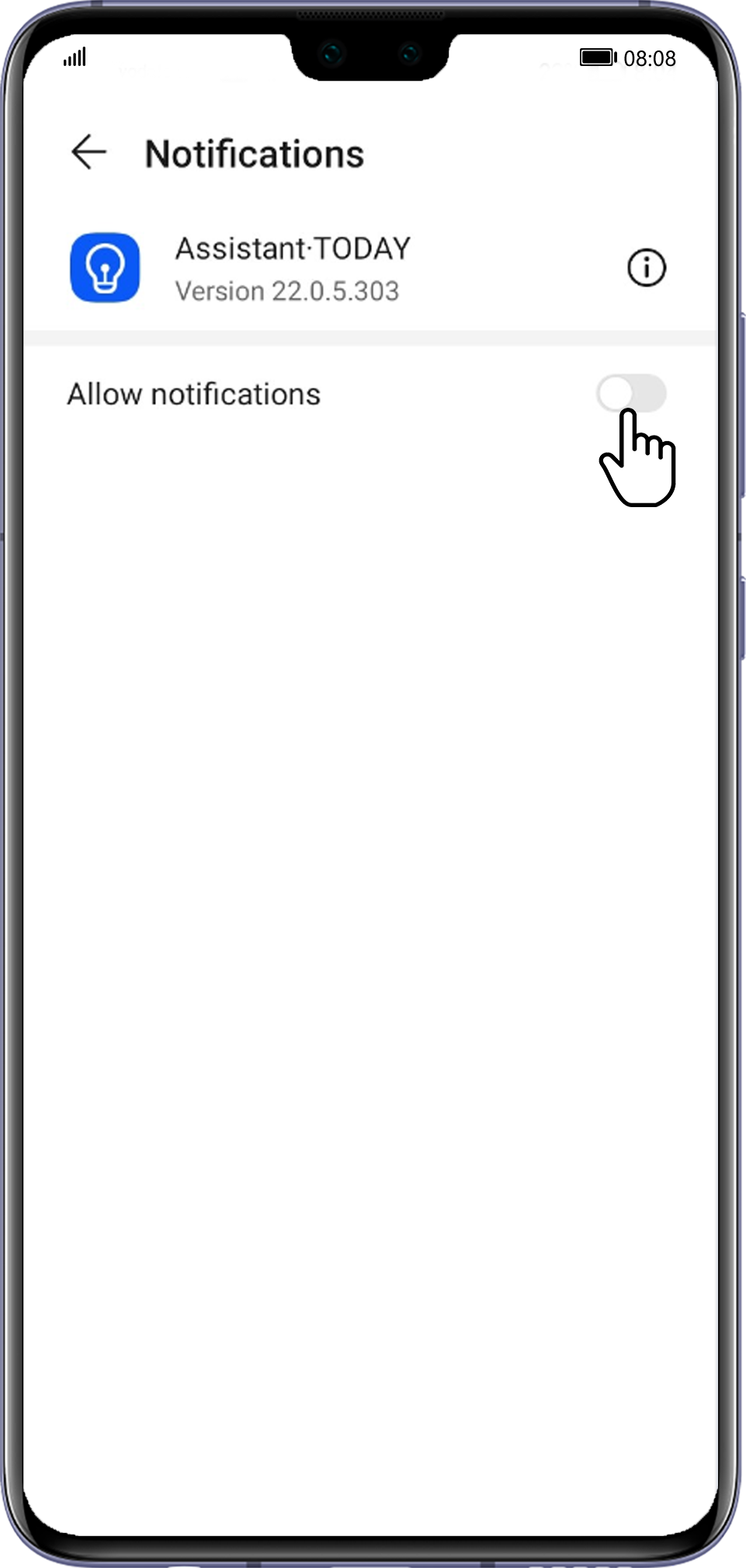The image depicts a smartphone screen displaying the "Notifications" settings for an app named "Assistant Today." The interface features a clean, white background. At the top, there's a navigation bar displaying "Notifications" with a left-pointing arrow for returning to the previous screen. Above this, the status bar shows five full signal bars, the time (08:08), and a full battery icon. The phone’s front camera, with two lenses, is also visible within the notch at the top center.

Beneath the navigation bar is the app's logo, consisting of a blue square with a white light bulb outline. The app version is listed as "Version 22.0.5.303" to the right of the logo. Next to this version information is an info icon—a black circle with a lowercase 'i'—which users can click for more details.

Underneath, there is a toggle option to allow notifications for the "Assistant Today" app, which is currently switched off. The user's cursor, customized to resemble a hand, hovers over this switch, indicating an intent to potentially enable notifications.

Surrounding the screen, the silver bezel of the phone is visible, with the volume buttons located on the right side alongside the phone's power button. The overall framing provides a clear depiction of the phone's physical attributes, emphasizing its sleek design.